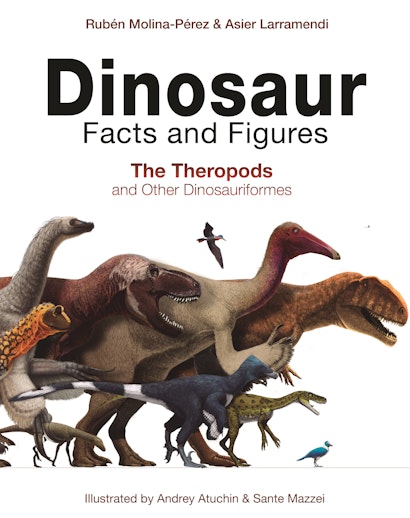The image depicts a book cover with a white background featuring detailed illustrations of various dinosaurs and a bird. At the top of the cover, the authors' names, Ruben Molina-Perez and Asier Laramendi, are prominently displayed in red text. Below this, in black text, is the title "Dinosaur Facts and Figures," followed by the subtitle in red, "The Theropods and Other Dinosaur Forms." The center of the cover showcases a vibrant array of around ten 3-D dinosaur illustrations, including species like T-Rex and Velociraptors, with a mix of brown and other colored dinosaurs. There's also a blue and white bird on the ground, suggesting the evolutionary link between dinosaurs and birds. At the bottom, in red text, it states, "Illustrated by Andrey Atuchin and Sante Mazzei."